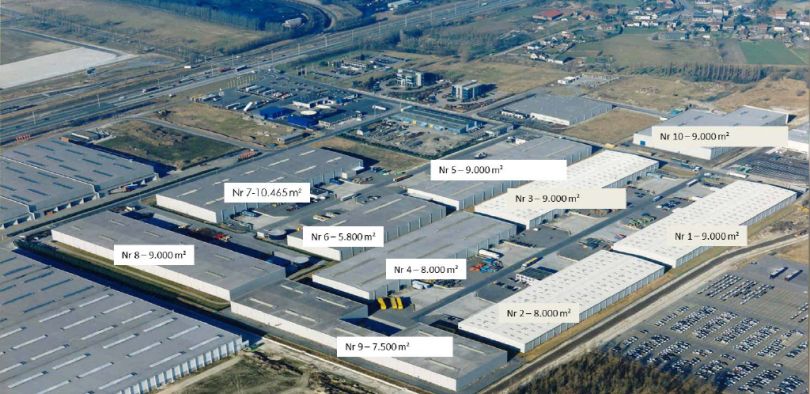This landscape-oriented aerial photograph, taken from a high-altitude drone, vividly captures an expansive industrial complex, likely located in the United States. The image focuses on a sprawling array of low-lying commercial-style buildings arranged in a roughly square formation, turned at an angle with its bottom edge near the center of the frame. These tightly packed structures dominate the scene, their flat, white or gray roofs suggesting modern construction methods. 

Overlaid text labels, in white rectangles with black text, are prominently displayed on the rooftops of most buildings. Each label features an 'NR' prefix followed by a number and the area size in square meters, such as NR-8, NR-7, and NR-6, with respective measurements like 9,000 m², 10,465 m², and 5,800 m². The exact significance of the 'NR' labels remains unclear but suggests a systematic identification method.

Adjacent to the buildings are several parking lots, with a particularly large one situated in the bottom right corner and another towards the middle. A major highway is visible beyond the complex on the top left of the photograph, alongside farther commercial areas, residential zones, and expanses of open fields, grounding the setting in a mixed-use landscape. The style of this image combines elements of representational realism with the precision of drone photography, highlighting both the industrial function and the extensive spatial planning of the area.